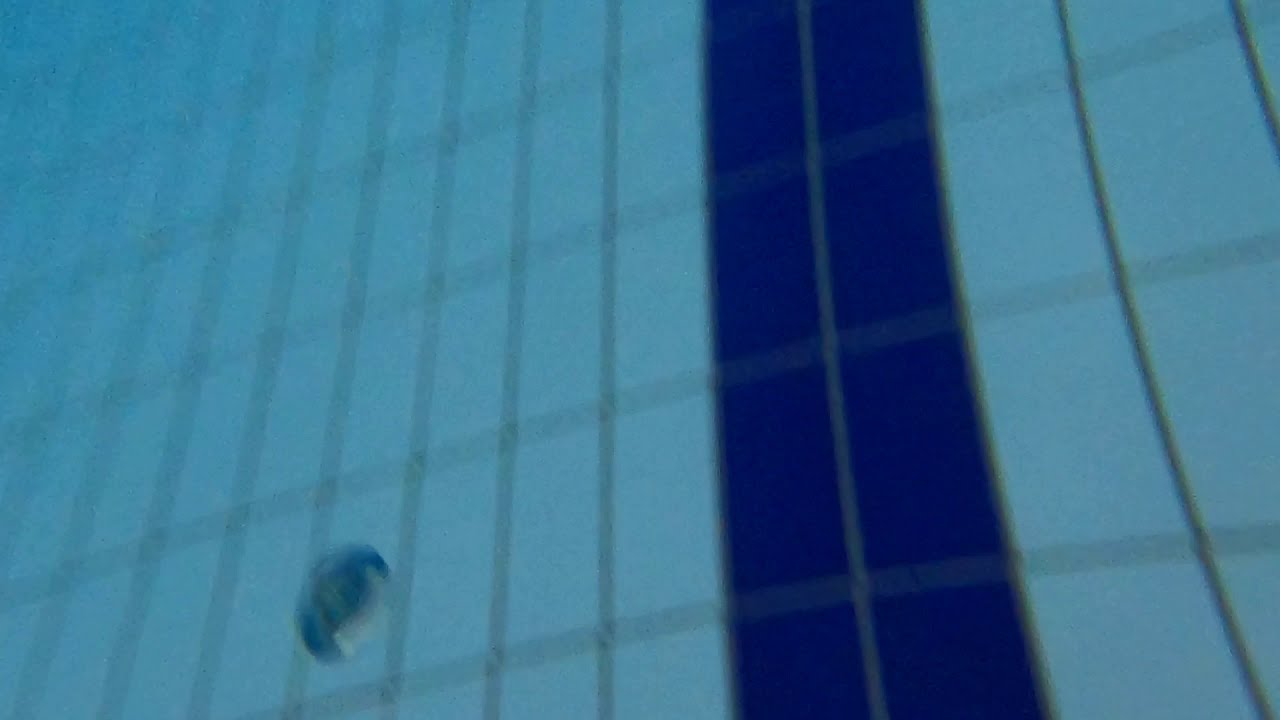The photograph presents an unfocused and slightly grainy underwater scene, likely the bottom of a swimming pool or hot tub, characterized by a grid of tiles. The tiles are primarily light blue or white in color, with two distinct dark blue tile stripes running vertically, slightly off-center to the right. These stripes are two tiles thick and contribute to the otherwise meticulous pattern of the tiles arranged horizontally and vertically. The image appears to be taken underwater, adding to the blurriness and making details less distinct. Towards the bottom left corner, a round blue object, possibly a drain or plug, can be spotted on one of the light blue/white tiles. The overall image has a blue tint and appears slightly tilted, becoming dimmer and foggier towards the left side.